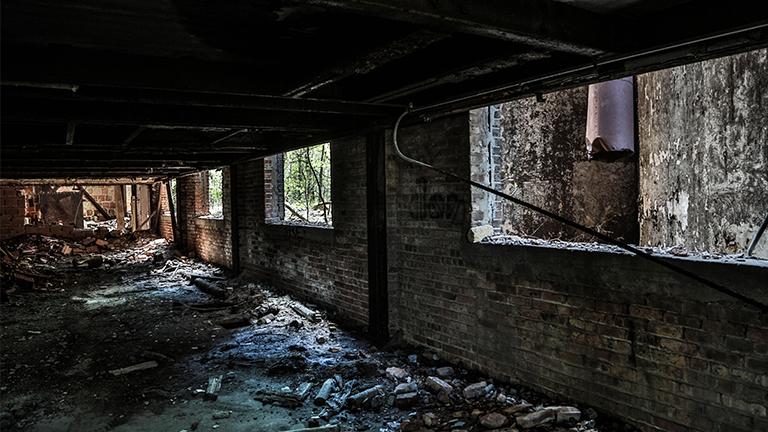In the image, we have a wide landscape perspective of the interior of an abandoned and severely worn-down old brick building, possibly a warehouse. Dominating the scene is a large brick wall on the right-hand side, which spans about 75% of the image before it transitions to the rear wall. The bricks, brown and worn, suggest the building has stood for over 50 years. This wall features several rectangular gaps where the windows once were; now, all of them are broken or knocked out, allowing views of an outside wooded area with visible trees. On the floor, there is a massive amount of scattered debris, including broken bricks and stones, all contributing to the impression that the building is in the midst of demolition or has been left to deteriorate over many years. At the top of the image and in the ceiling area, there are blackened or charred beams, indicating that a fire might have ravaged the structure at some point. The center and left side of the image reveal further piles of rubble, adding to the chaotic and abandoned nature of the scene. Light filters into the space through the broken windows and a gap in the ceiling on the left, illuminating this relic of a bygone era.